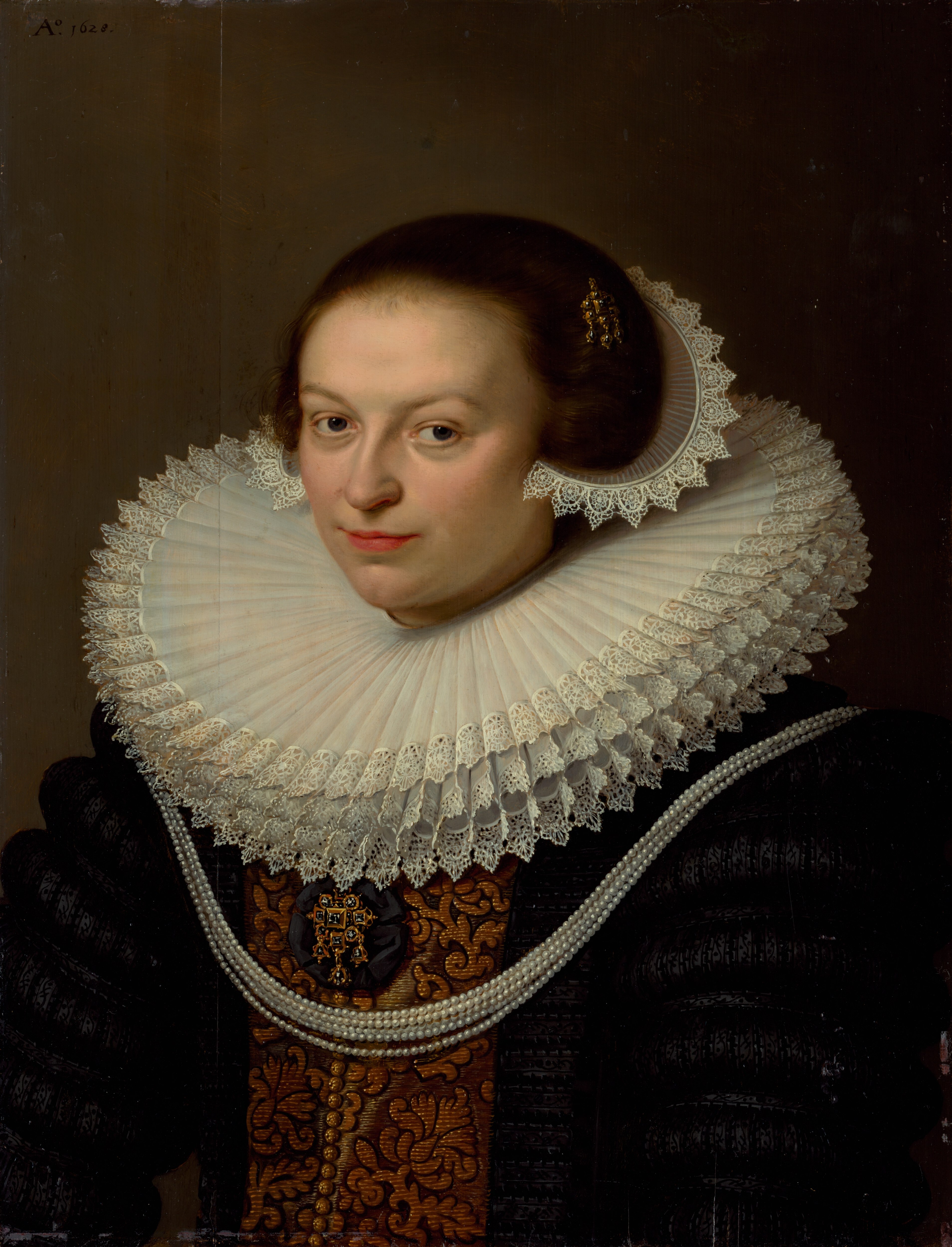This is a detailed portrait of a middle-aged queen, likely from the 15th to 17th century, depicted in royal attire against a dark brown background. Her hair is neatly pinned back and adorned with a diamond-encrusted crown and a decorative hairpiece. Around her neck, she wears a prominent white, layered, floofy lace collar, which further accentuates her royal bearing. Draped gracefully from her shoulders and curving beneath her chin are several strands of pearls, showcasing her elegance. She dons an intricate black gown with a brown center line running vertically from under her neck to the bottom of the painting, featuring buttons and intricate designs. The central brooch on her dress adds to the garment's opulent details. She has a fair complexion, a wry smile, and her lips are adorned with lipstick as she gazes directly at the painter, exuding regal poise and dignity.